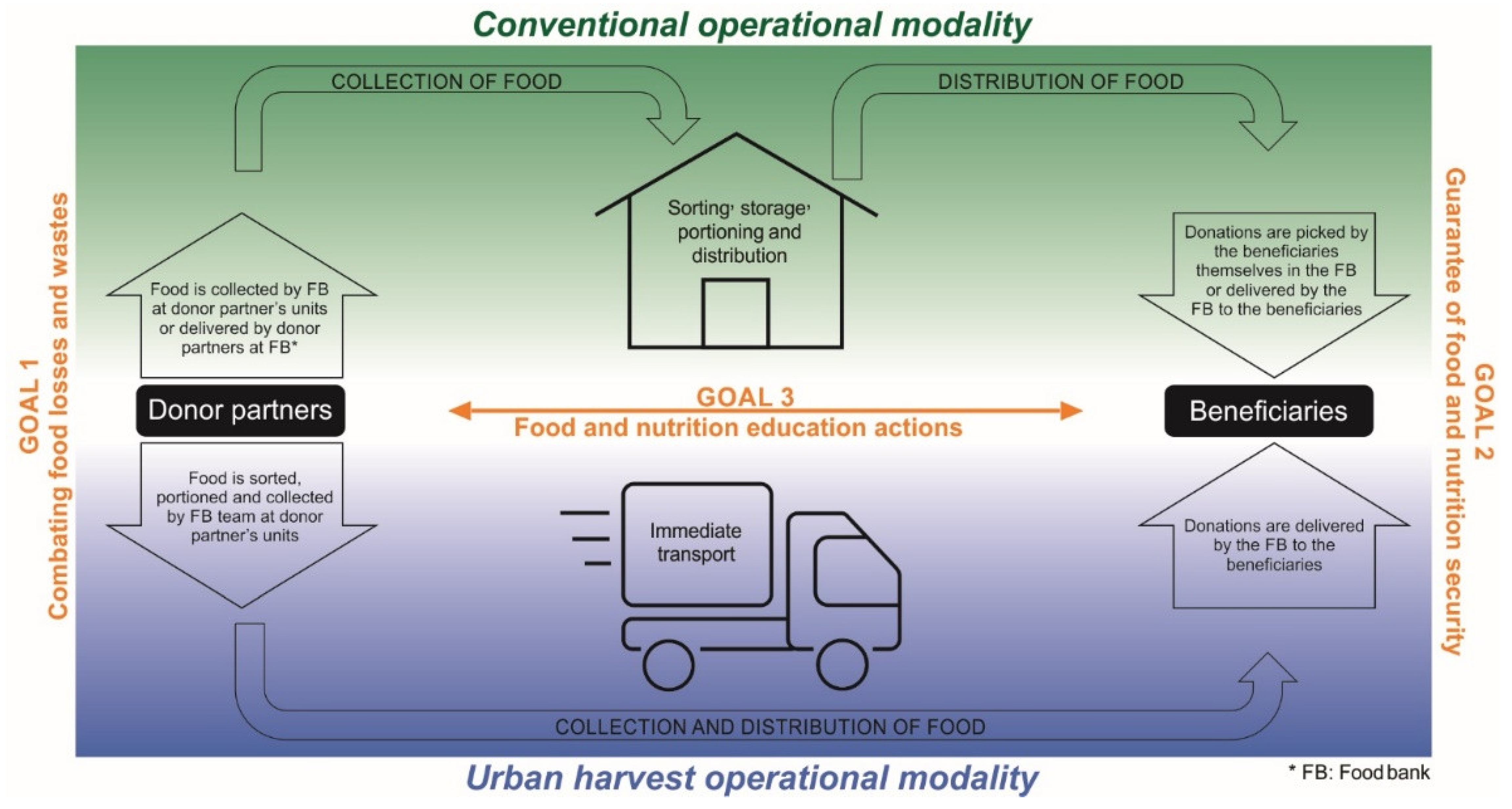The image displays a detailed flowchart titled "Conventional Operational Modality," illustrating the processes of food collection, sorting, distribution, and education by a food bank. The chart is structured to highlight two main goals: Goal 1, "Combating Food Losses and Waste," on the left, and Goal 2, "Guarantee of Food and Nutrition Security," on the right, alongside an overarching Goal 3, "Food and Nutrition Education Actions."

Starting from Goal 1, food is collected by the food bank (FB) either at donor partners' units or delivered to the FB by donor partners, represented by a black box with white lettering. This process is shown with a chunky arrow leading to a house-like symbol indicating sorting, storage, portioning, and distribution. A skinny arrow follows, pointing toward the distribution phase where food is either picked up by beneficiaries at the FB or delivered to them by the FB, illustrated by another chunky arrow labelled accordingly.

The diagram emphasizes the role of immediate transport, depicted with a truck icon located mid-chart, and the continuation of food distribution. An additional long skinny arrow named "collection and distribution of food" connects from the donor partners to the final distribution stage, integrating the truck symbol to highlight the logistics involved.

In the center of the poster, a prominent orange arrow labeled Goal 3 points towards both donor partners and beneficiaries, emphasizing the importance of food and nutrition education actions.

Visually, the chart is divided into green sections at the top where collection processes are detailed, and purple sections at the bottom indicating distribution stages, creating a clear, easy-to-follow flow for the viewer. The overall design efficiently communicates how food, initially collected from donors, is processed and eventually distributed to beneficiaries, aiming to prevent food waste and ensure nutritional security.